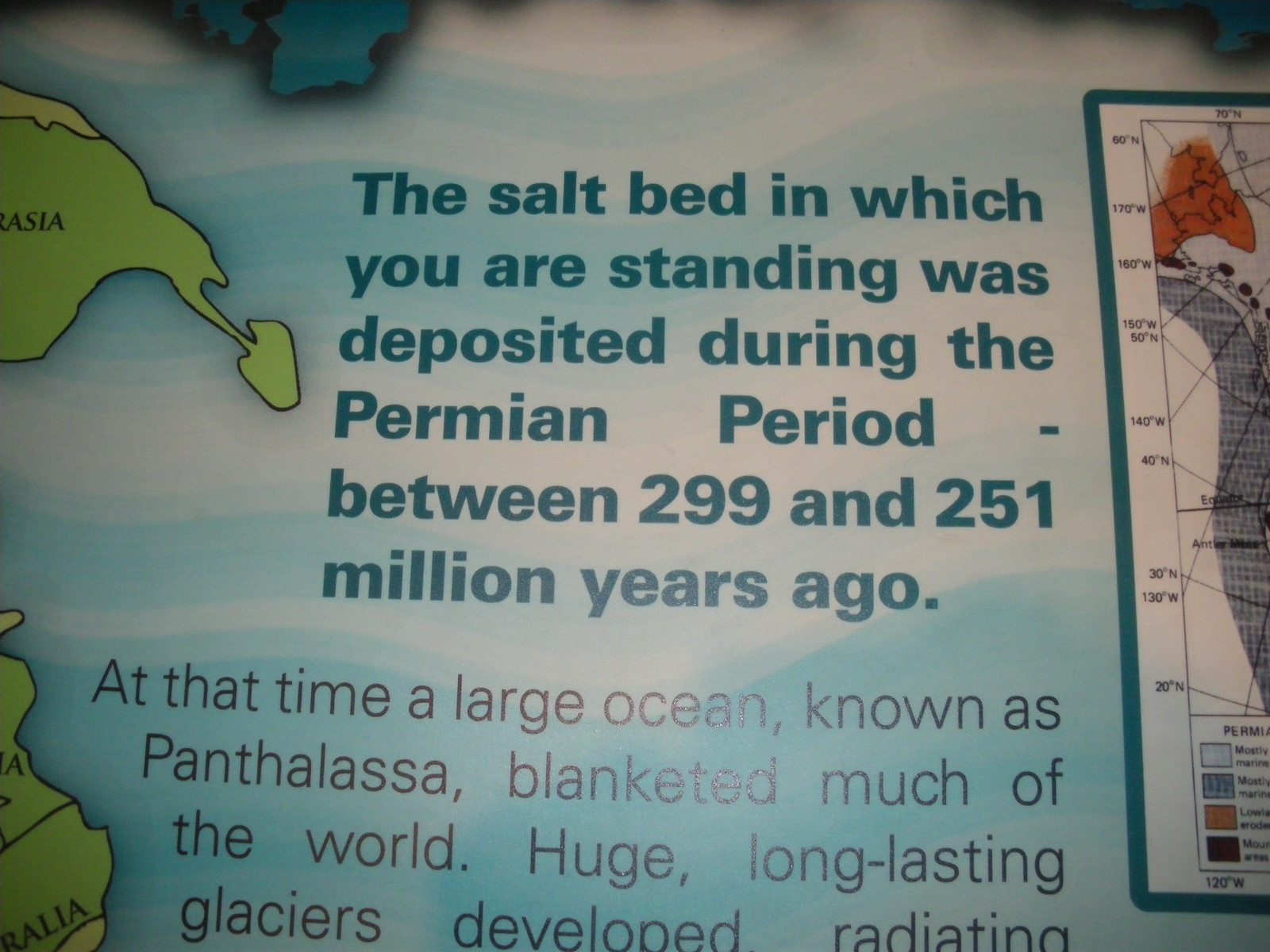The image showcases an up-close photograph of an informational sign, approximately six inches wide and five inches tall. The sign has a bluish-white background adorned with horizontal wavy white stripes blending into the blue. The main text, displayed prominently in bold blue font in the center, reads: "The salt bed in which you are standing was deposited during the Permian period between 299 and 251 million years ago." Below this, in black text, it states: "At that time, a large ocean known as Panthalassa blanketed much of the world. Huge, long-lasting glaciers developed, radiating," after which the text is truncated.

To the left of the sign, there is an image of Asia colored in green, serving as a geographical landmark. On the right-hand side, there is a white rectangle with a blue border, containing graphical information of different terrains or mapping, which is partially out of view. This sign appears to be the type one might find in a museum or a park, providing historical and geological context for the location.